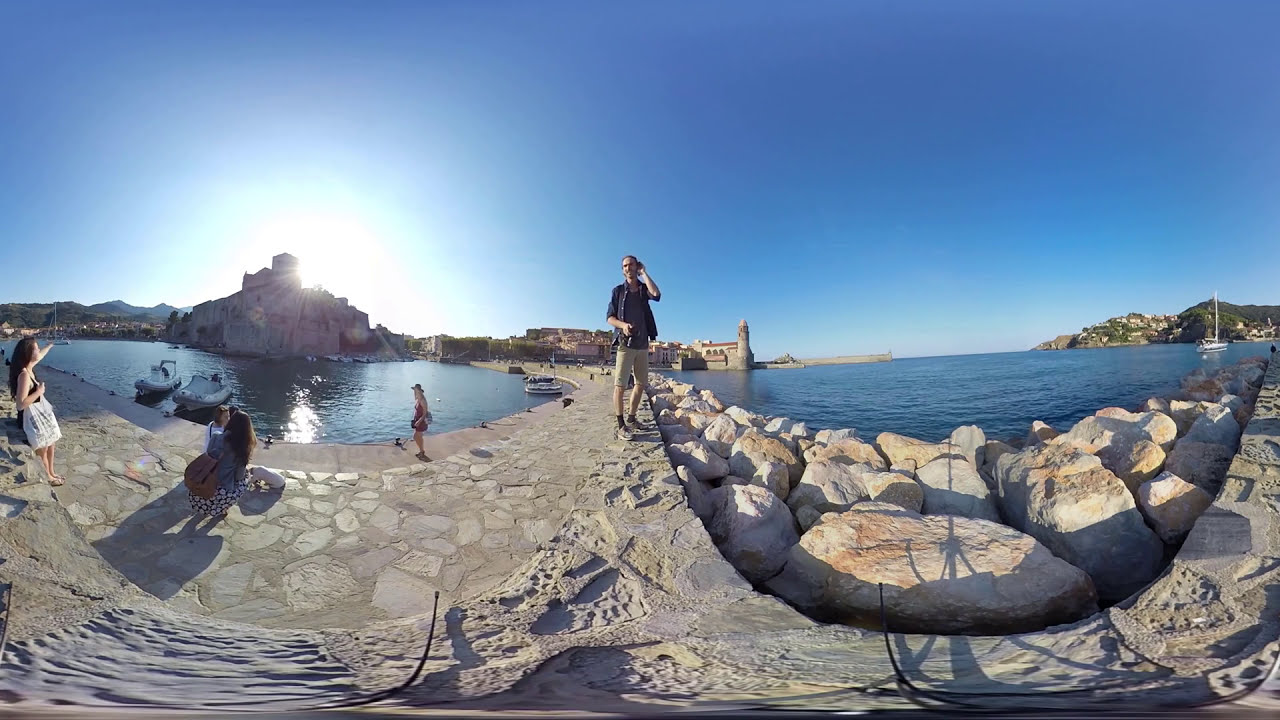This vibrant, sun-drenched photograph captures a lively seaside scene on a bright, cloudless day with a dazzling cobalt blue sky. Dominating the foreground is a stone-paved walkway where people, standing and sitting, glance out over a tranquil turquoise waterway that spans both sides of the path. The central figure, whose gender is indistinct, dons tan shorts and a dark blue t-shirt. With one arm bent and the forearm slightly extended and the other reaching up to the side of their head, they seem to be engaging with a device, possibly a phone.

To the left of this central figure, a woman with long brown hair, wearing a sleeveless top and carrying a tote bag, stands near a child who appears to be engrossed in some activity at the water's edge, possibly feeding ducks or sea life. Further along on the left, a person, perhaps in a bathing suit, walks a small dog on a leash.

On the right side, the waterway continues, bordered by large stone boulders. At the far right of the image, a docked sailboat with its mast standing bare is visible. In the distance, a rocky, hilly landmass stretches toward the horizon, adorned with a series of buildings that resemble an old lighthouse or fort. Among these, a prominent structure stands out — it has the appearance of a castle or an ancient church, its brick façade and tall spire casting long shadows in the brilliant sunlight.

The photograph's overall atmosphere is serene, capturing the leisurely activities of visitors against the backdrop of a pristine, clear waterway and striking historic architecture, all bathed in the golden glow of a perfect day.